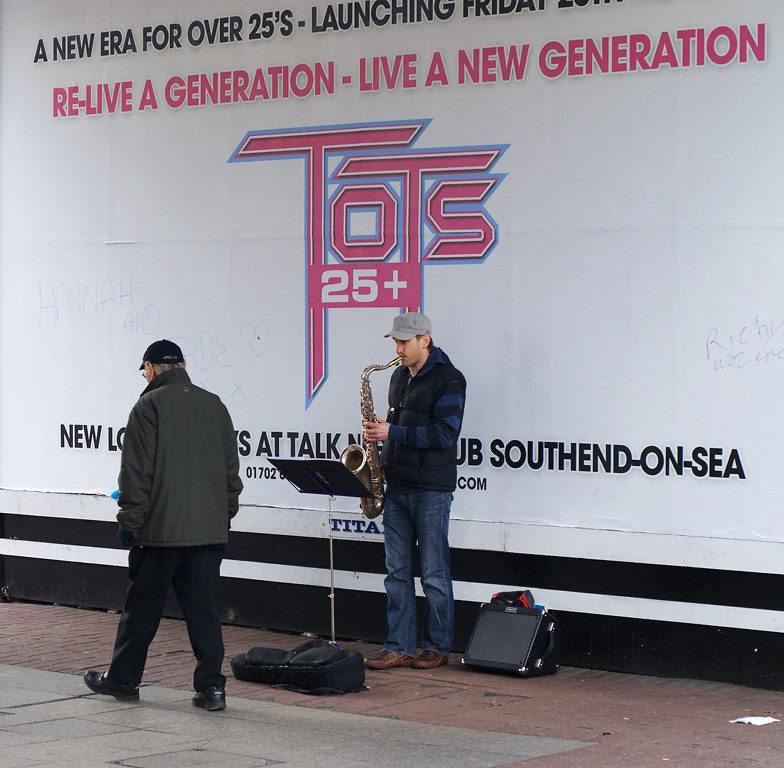In this detailed image, a man is playing a tenor saxophone outdoors in front of a white billboard. The billboard prominently displays phrases such as "A New Era for Over 25s," "Launching Friday," "Relive a Generation, Live a New Generation," and "Tots 25+," with the latter in pink and white text. The bottom part of the billboard has more text, including "South End on C," partially obscured by two individuals.

The saxophonist, a white male, sports a gray baseball cap and a navy blue life preserver-style vest over a striped blue shirt. He also wears blue jeans and brown boots. Positioned before him is a music stand holding sheet music, and at his feet is a soft saxophone case, suggesting he is busking. An amplifier is placed on his left, enhancing his performance.

To the left, an older man, possibly in his 70s, walks past, facing away from the camera. He's dressed in a gray jacket, black pants, black shoes, and a black hat, with gray hair peeking out. The sidewalk beneath them is a mix of red brick and gray concrete, adding a textured contrast to the scene.